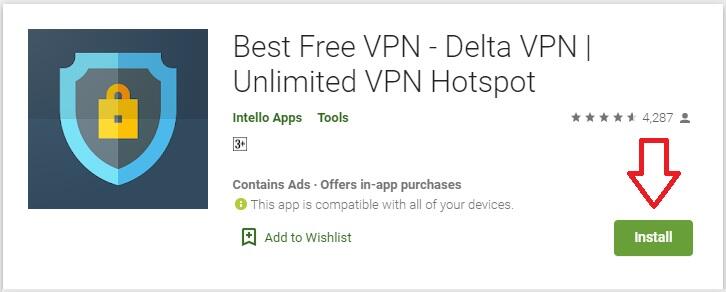The image features a large white rectangle bordered in light gray, adorned with very thin black lettering. At the top, it reads "Best Free Capital VPN - Delta Capital VPN," followed by a dividing line. Beneath this, in capitalized black lettering, is "Unlimited VPN, Hotspot." Below this, in a bold mossy green font, the text "Intello Apps" appears, followed by a space and then "Tools." To the right of this section, a user rating of approximately 4.5 out of 5 stars is displayed alongside the number "4,287" and a user icon.

Directly under the "Intello Apps" text, there is a bold black "3+" within a square, indicating the app's rating. Below this, in bold gray lettering, it states "Contains Ads," followed by a bullet point and "Offers in-app purchases." Beneath this, in non-bold font, it mentions, "This app is compatible with all of your devices." To the left of this sentence is a circular icon filled with green, featuring a white eye, symbolizing information. Below this section, there is a tag symbol with a plus sign accompanied by the text "Add to Wishlist," displayed in green with the tag symbol in dark green and bolded.

The app's icon, positioned towards the left, is rather large and square-shaped, divided into four sections with varying shades of navy blue. It depicts a shield outlined with a thick light blue border, shaded in gray-blue color, featuring a gold padlock at its center.